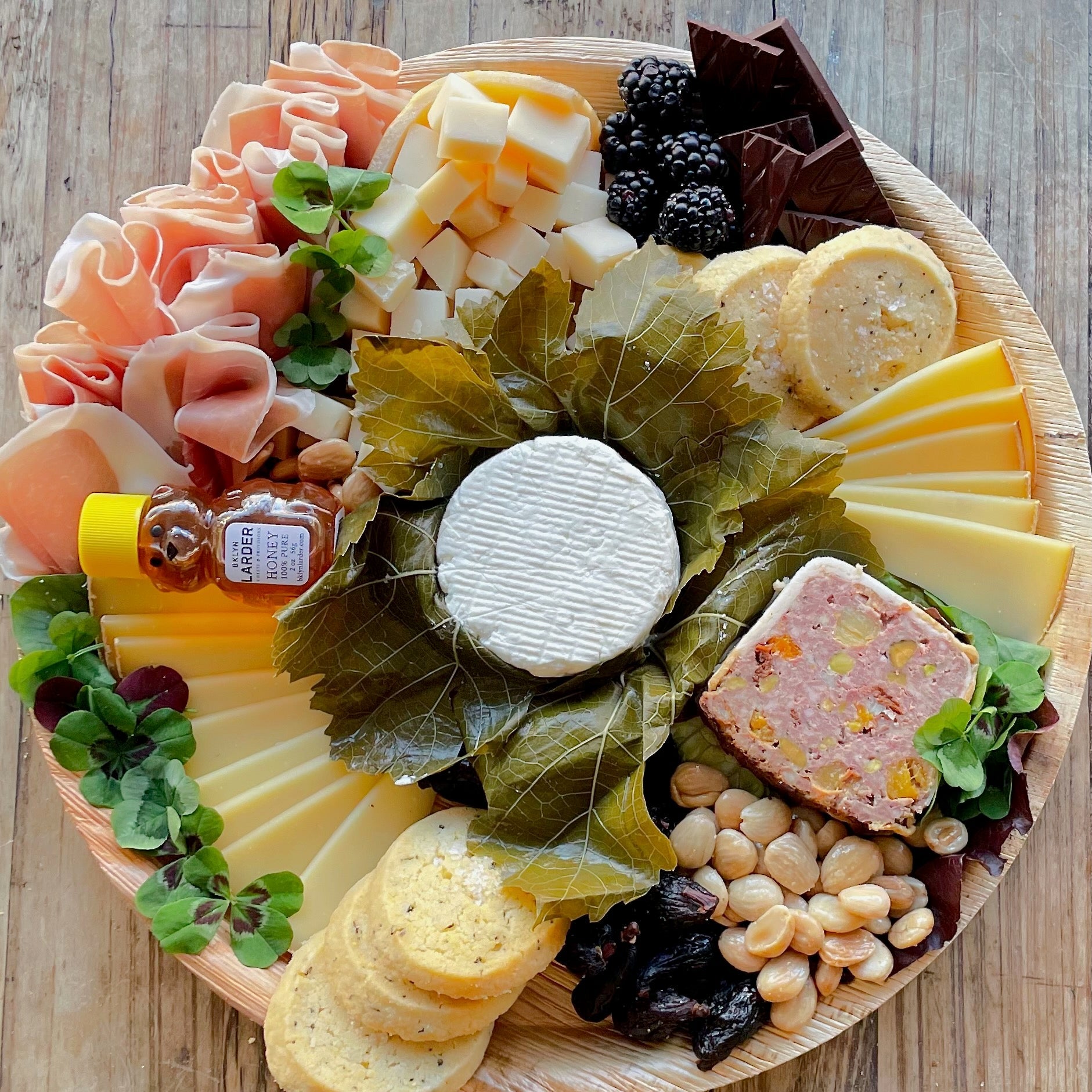This overhead photograph beautifully captures a meticulously arranged round charcuterie plate, positioned on a weathered wooden surface resembling a picnic table. The light brown, wooden grained plate showcases an array of delectable items. At its center lies a round, soft, white cheese nestled in a bed of large green grape leaves. Surrounding this centerpiece, an artistic spiral arrangement features a variety of lunch meats, an assortment of cheeses, blackberries, pieces of dark chocolate, a small bear-shaped bottle of Larder Honey, green clovers or decorative accents, nuts, dried fruits, and plenty of crackers. Every item is placed with care to create a harmonious and visually appealing presentation, highlighting the fresh and delicious contents of the charcuterie board.